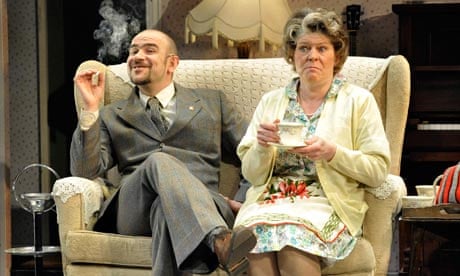In this vibrant photograph, reminiscent of an endearing sitcom scene, a man and a woman sit closely on a cream-colored loveseat adorned with a matching throw draped over its back. The man, dressed in a sharp gray suit, sports a well-groomed beard and a goatee. He exudes confidence as he smiles warmly, legs crossed, with one elbow propped on the arm of the loveseat. His animated expression is accentuated by his hand raised mid-gesture, likely emphasizing a jovial or important point.

Beside him, an older woman, exuding a matronly charm, presents a stark contrast. Dressed in a modest dress paired with a cardigan and an apron tied meticulously around her waist, she clutches a delicate teacup and saucer. Her elaborate short gray hair frames a face etched with distress, her wide eyes and furrowed brows capturing an expression of alarm. This contrast between the man’s relaxed demeanor and the woman’s evident concern creates a dynamic and engaging visual narrative.